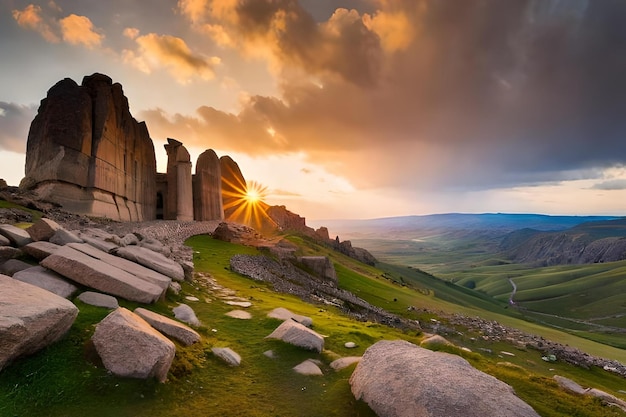This detailed horizontal, rectangular-shaped photo showcases a stunning rural landscape of rolling hills and vast grassy areas, peppered with a multitude of rocks and imposing boulder formations. The terrain is far from flat, with giant rock formations standing prominently and casting shadows that suggest the setting or rising sun is near. The sky is adorned with a mixture of dense clouds and clear patches that seem to suggest an overcast atmosphere, though the sunlight creates dramatic visual effects. The scene is framed with green grass and rocky hillsides extending into the background, primarily to the right. Despite its natural look, the light and color scheme have an almost otherworldly quality, suggesting a possible computer-generated enhancement. The untouched and expansive land hints at an area far removed from urban development, capturing a timeless and serene beauty.